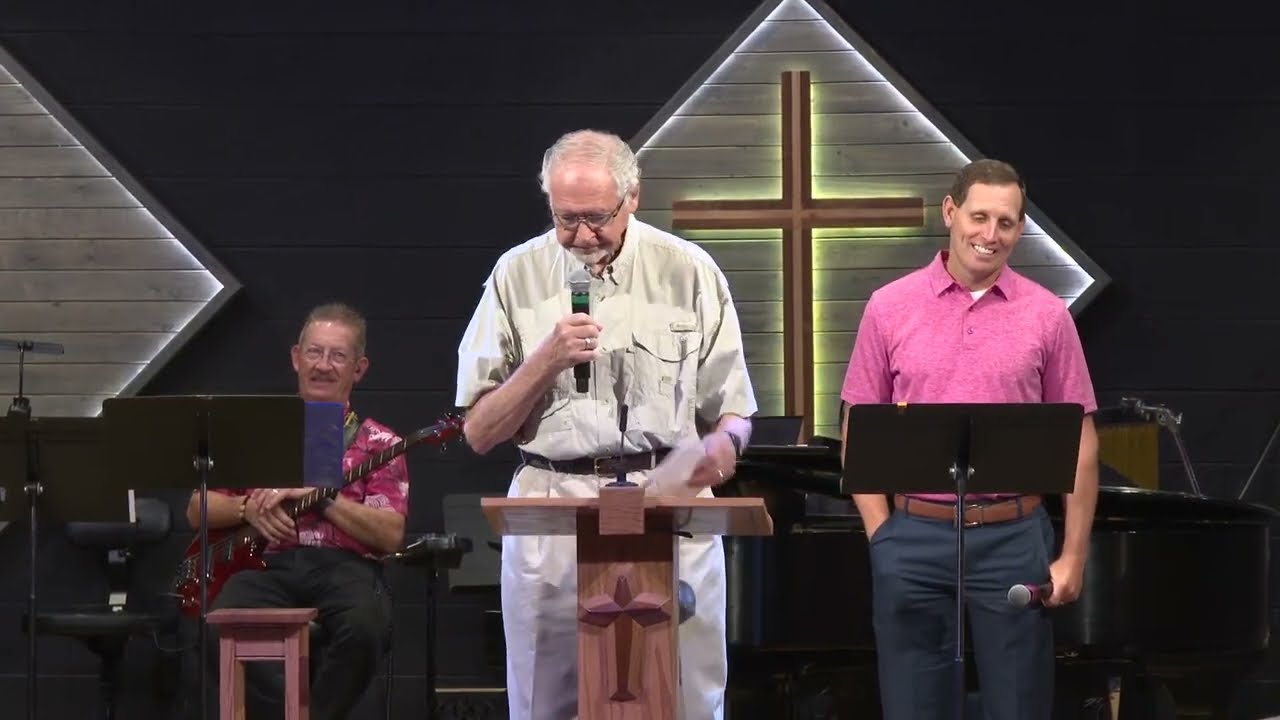This detailed color photograph captures a moment indoors at a church during what appears to be a religious event. In the center, an older gentleman stands at a wooden podium bearing a cross emblem. He has thinning gray hair, fair skin, and wears glasses. Dressed in a white button-up short-sleeved shirt, white pants, and a brown belt, he holds a black microphone with a silver top and a green band below the top in his right hand, while his left hand holds a piece of paper. He is looking down as he speaks into the microphone.

To his left, an older man with white hair, wire-rimmed glasses, and a mustache sits, holding a red electric guitar across his chest. He wears a red-flowered shirt and gray slacks. In front of him stands a music stand, possibly accompanied by a microphone or cymbals to his left.

On the far right stands a younger man with short brown hair, dressed in a short-sleeved pink collared shirt, gray slacks, and a brown belt. He looks down at a music stand in front of him and smiles, also holding a microphone down at his side.

The background features a gray cement stone wall with two wooden triangular elements. In the center triangle stands a large illuminated wooden cross. The overall composition reflects a serene and dignified atmosphere, characteristic of a church setting.